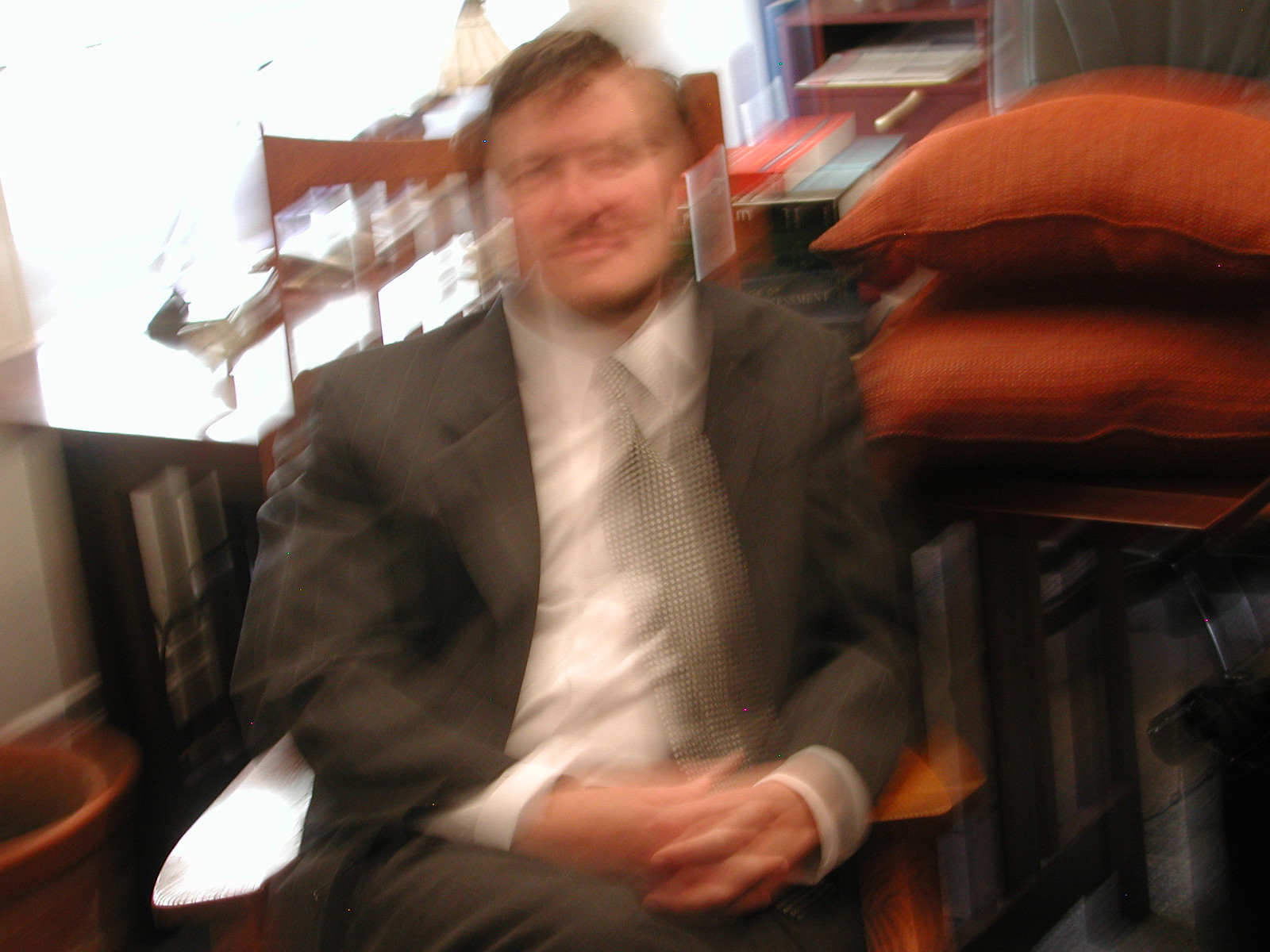In the image, there is a very blurry front-view picture of a man dressed in a suit. The man, appearing older with short brown hair, is seated with both arms drawn inward, interlocking his hands on his lap. Despite the blurriness, his face is faintly visible, showing a slightly smiling expression without any teeth showing. He is clad in a suit that is a brownish-dark gray color, paired with a white undershirt and what seems to be a gray tie, though the blurriness gives the illusion of multiple ties. The suit’s collars and the sleeves are white. His pants are also brown. Behind the man, there are two orange pillow cushions situated on the top right of a brown table. The background also features a couple of books and a prominent white light shining from the left-hand corner.